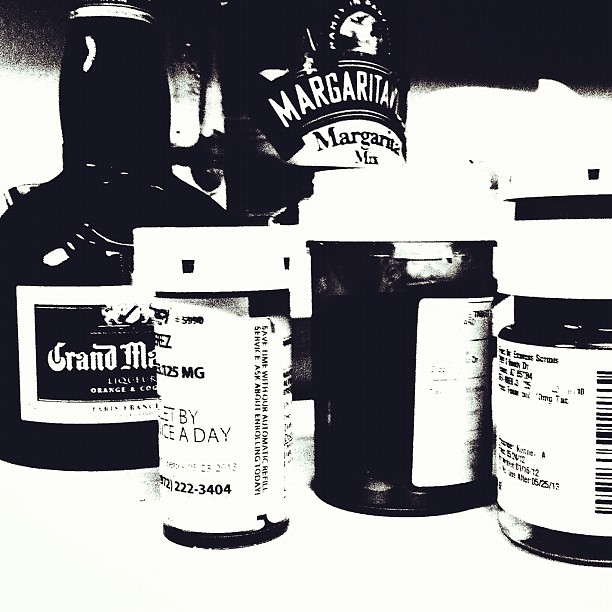The black and white photograph is artistically styled, capturing an array of contemporary items that blend the medicinal with the recreational. Dominating the top left, a 750 milliliter bottle of Grand Marnier liqueur, distinguished by its unique shape, proudly displays "Grand Marnier," "liqueur," and "orange" in white font on a dark label. To its right, a larger margaritamix bottle stands tall, adding to the visual depth. Below these, in the forefront of the image, sit four pill bottles of varying sizes and shapes, each meticulously detailed with labels and safety caps. The first pill bottle on the left, partially turned, reveals text indicating dosage and a fraction of a phone number, "222-3404". The bottles are characterized by their darker hues with stark white caps and labels, inscribed with black writing. The middle pill bottles display intricate details such as "125 milligrams" with instructions about daily intake, while another, resembling a vitamin bottle, features a visible barcode. The whole image is devoid of color, enhancing its artistic appeal and drawing attention to the contrast and textures of the objects on display.